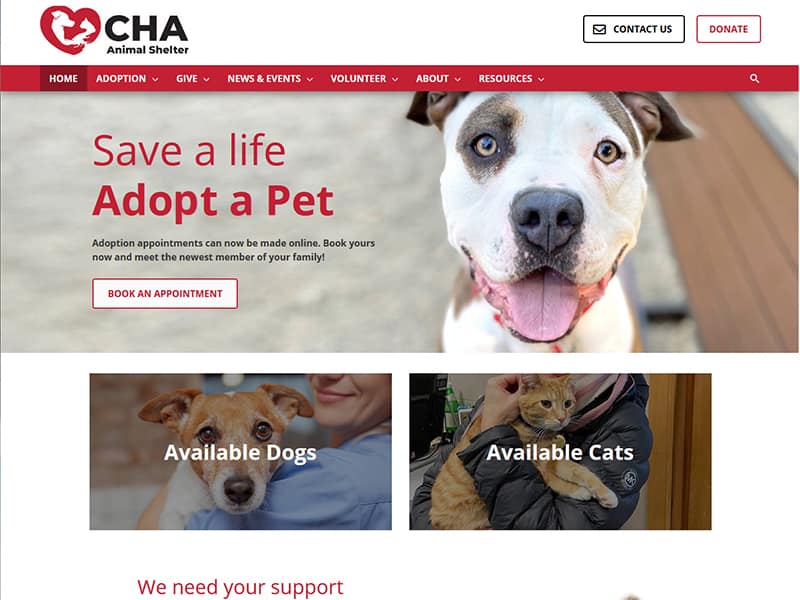On a clean white background, the image features a black and white logo of an animal shelter. At the center, there is a red heart enclosing silhouettes of two animals, likely a cat and a dog. The top part of the image includes a black rectangle with the text "Contact Us" next to an envelope icon. Adjacent to this, a red rectangle reads "Donate," while the word "Home" is highlighted against a burgundy background, indicating it is selected. Additional navigation options include "Adoption," "Give," "News and Events," "Volunteer," "About," and "Resources," with a magnifying glass icon located on the far right for search functionality. 

Prominently displayed, the phrase "Save a Life. Adopt a Pet." accompanies an image of a playful puppy with a brown spot on its eye, its tongue hanging out. Below the main phrase, text informs that adoption appointments can now be made online, encouraging viewers to "Book yours now and meet the newest member of your family." A red button on a white rectangle prompts "Book an Appointment."

Further sections highlight "Available Dogs," illustrated with a picture of a woman holding a dog, and "Available Cats," depicted by what appears to be a woman holding a cat. Notably, in red text, the image conveys a call to action: "We Need Your Support."